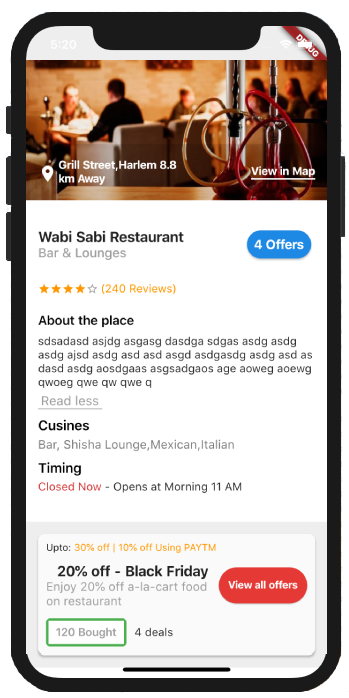A screenshot from a mobile app showcases a Wasabi Restaurant Review. The image captures the ambiance of the Wasabi Restaurant, a bar and lounge situated on Grill Street, Harlem, approximately 8.8 kilometers away. The photograph is taken from the vantage point of the bar, focusing on the bar tabletop while the patrons in the background are slightly blurred. Two individuals are seen sitting at a table under soft lighting, possibly emanating from a skylight. The restaurant’s interior decor is accentuated with hues of brown, red, gray, and tan. Adorning the upper walls are framed pictures, contributing to the cozy yet sophisticated atmosphere. 

Detailed information on the app indicates the restaurant’s multifaceted cuisine, featuring offerings from the bar, sushi, lounge, Mexican, and Italian. Although currently closed, the establishment opens at 11:00 AM on Monday morning. The app lists four enticing offers, including a notable 20% off for Black Friday, with an option to view all available deals. The user interface prominently displays these details, making it convenient for users to explore the restaurant’s offerings and plan their visit.